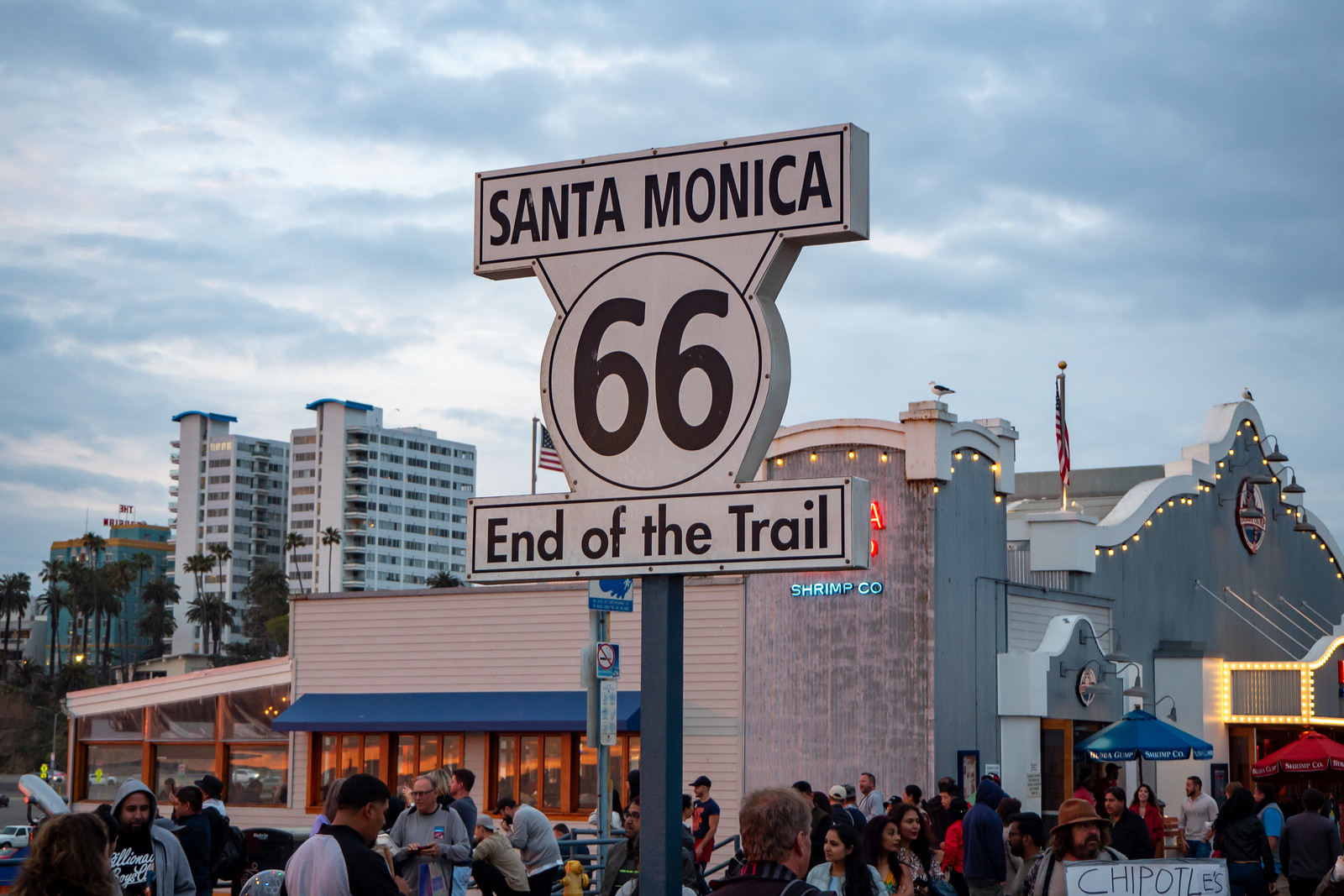This horizontally oriented rectangular photograph captures a bustling scene at the iconic Santa Monica boardwalk in California. Dominating the foreground is a white sign mounted on a gray metal pole, centrally positioned in the image. The sign features two white rectangles—one at the top with "SANTA MONICA" in bold black letters and one at the bottom with "END OF THE TRAIL" also in black. Between these rectangles, a white circle showcases the bold black number "66," signifying the end of the historic Route 66.

Above the sign, the top half of the image reveals a mostly cloudy sky, with gray clouds interspersed with patches of white where the sun tries to break through, suggesting a late afternoon setting. Behind the sign lies a lively crowd of people walking and socializing, presumably enjoying their time on the boardwalk and near local establishments.

In the background, a commercial building with a distinct curved wall made of gray stone is partially visible. The building features illuminated blue letters spelling "Shrimp Company," likely referring to the famous Bubba Gump Shrimp Co. restaurant, while red letters above are obscured by the sign. Beyond this, an American flag flutters, and several tall, condo-style buildings rise against the skyline, adding to the urban backdrop. The overall scene is rich with colors including gray, white, blue, red, and shades of orange and brown, evoking a vibrant and dynamic outdoor atmosphere.